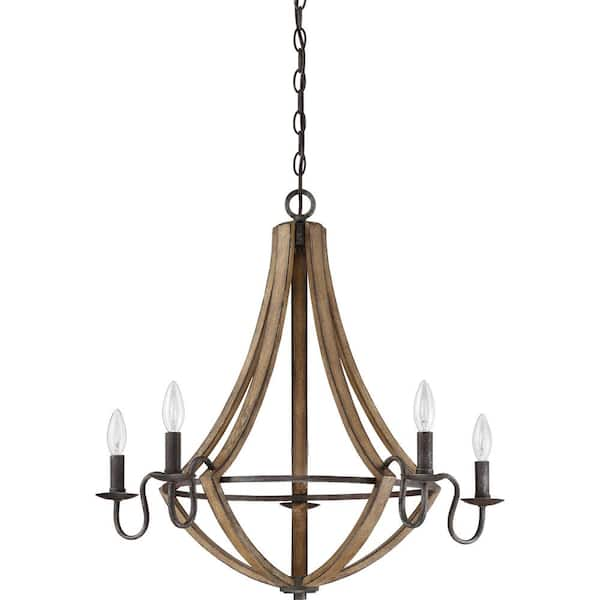The image features a chandelier suspended from a ceiling by a brown cord encased in a circular chain. The background appears as a blank, white expanse, offering no additional context. The chandelier's main structure begins with a single wire running down from the ceiling, adorned with four evenly spaced black rings closely aligned along the wire. Just before the wire meets the chandelier's primary body, a larger black ring is positioned horizontally, facing the viewer.

The body of the chandelier consists of several distinctive elements of burnished brass. From a central vertical cylindrical rod, four thin brass arms extend outward in an equilateral layout, bending back towards the center about two-thirds of the way down. These arms then rejoin at a bottom black ring, creating a cohesive, circular arrangement.

Attached to this bottom ring are four black metal rods, which curve outward before supporting the light fixtures. Each fixture holds a black socket that houses a narrow bulb reminiscent of a flame, encased in clear crystal glass. The bulbs are designed to mimic the shape of a flame, adding a decorative and elegant touch. The overall aesthetic combines black metal and burnished brass elements, producing a sophisticated appearance.